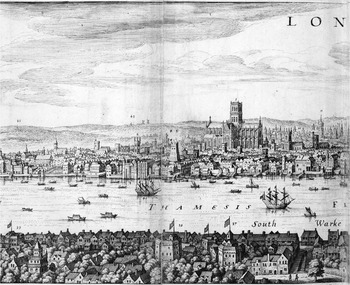This vintage black-and-white image, resembling an old map or print, appears to be a detailed drawing taken from a book. The binding curve at the center indicates it spans across two pages. At the top right corner, partially cut-off letters L-O-N suggest it depicts London. The centerpiece of the drawing is the River Thames, running horizontally from left to right, and crowded with various ships and boats, indicating a bustling waterway.

In the foreground, the city's skyline is intricately detailed with small houses and towers leading up to more prominent structures. The background showcases taller buildings, including impressive castles and a large church. The labels "Thames" on the river and "South Work" likely point to Southwark, a notable area in London. The scene is rendered in black ink or pencil, enhancing its historical and timeless feel, capturing a densely constructed urban area along the riverbanks.